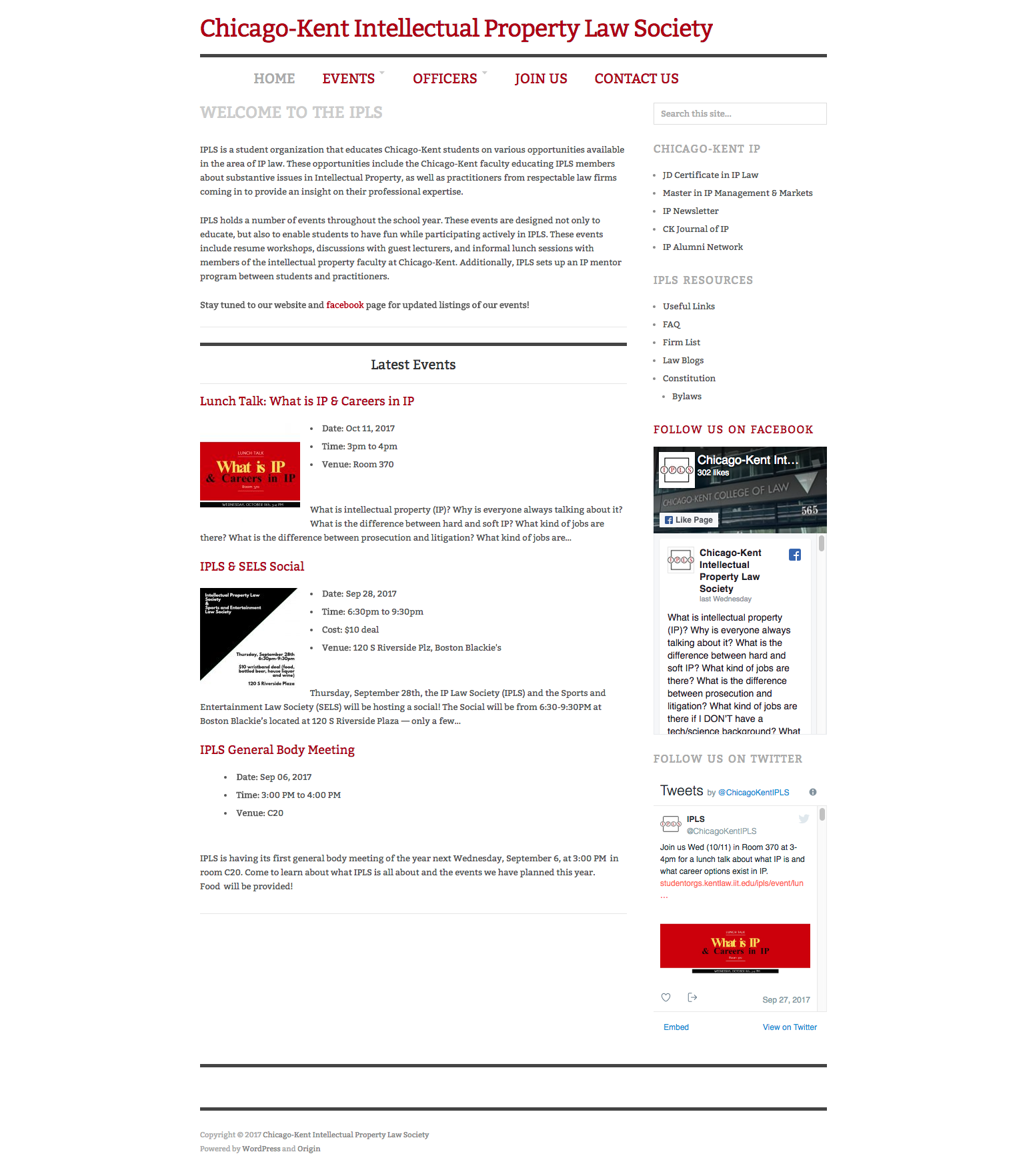The screenshot depicts a website viewed on a smartphone, evident from its narrow width and extended length. The background of the site is predominantly white. At the very top sits the headline in maroon font, reading "Chicago Kent Intellectual Property Law Society." Directly beneath this headline is a thin black line, followed by a horizontal navigation menu written in gray. The menu items include "Home," "Events," "Officers," "Join Us," and "Contact Us," with the latter four standing out in capitalized maroon font.

Further down, on the left side of the page, a light gray sub-headline welcomes visitors with the text "Welcome to the IPLS." Below this are two paragraphs of text, though the font size is too small to discern their content.

A black line separates these introductory paragraphs from the next section, labeled "Latest Events." This section features a maroon-colored rectangular banner with the text "What is IP?" in yellow font. The description beneath this banner is also too small to read.

On the right side, a sidebar occupies the length of the page, with a notable feature halfway down: a small screenshot from the organization's Facebook page. Above this image is the prompt, "Follow us on Facebook."